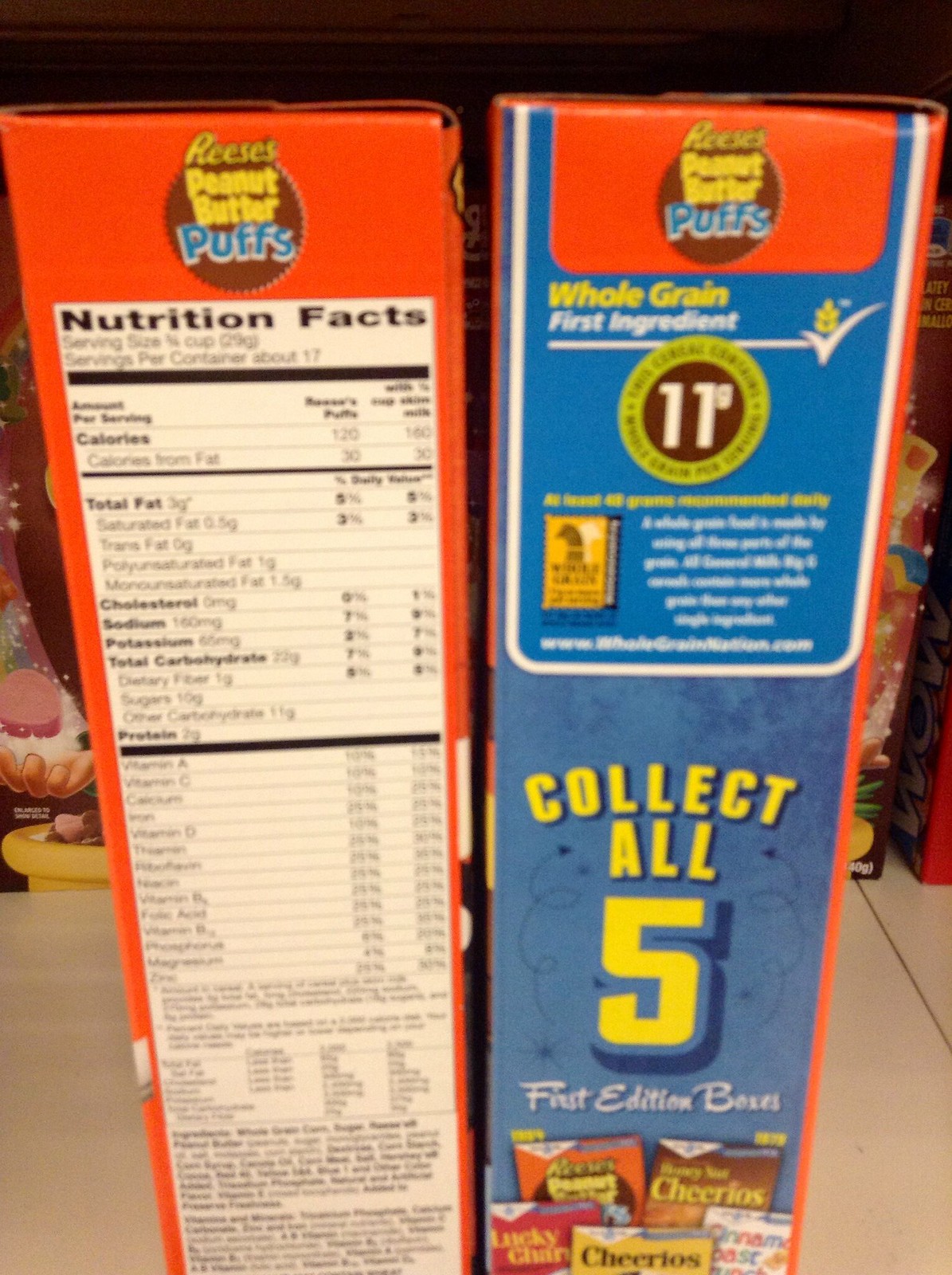A vibrant color photograph captures a scene in the cereal aisle of a grocery store, zooming in on two boxes of Reese's Puffs cereal placed side by side. The box on the left prominently displays the nutrition facts, though the text appears slightly blurry. Adjacent to it, the right box showcases an advertisement that reads "Reese's Puffs, whole grain, first ingredient." The text underneath is partially illegible due to blurriness, but the box also flaunts a collectible aspect, encouraging shoppers to "collect all five first edition boxes." Alongside this message, small images of other cereals such as Lucky Charms, Cheerios, Cinnamon Toast Crunch, and Honey Nut Cheerios can be seen at the bottom. Both boxes rest on a store shelf, with parts of other cereal boxes visible in the background, contributing to the lively, bustling ambiance of the grocery aisle.